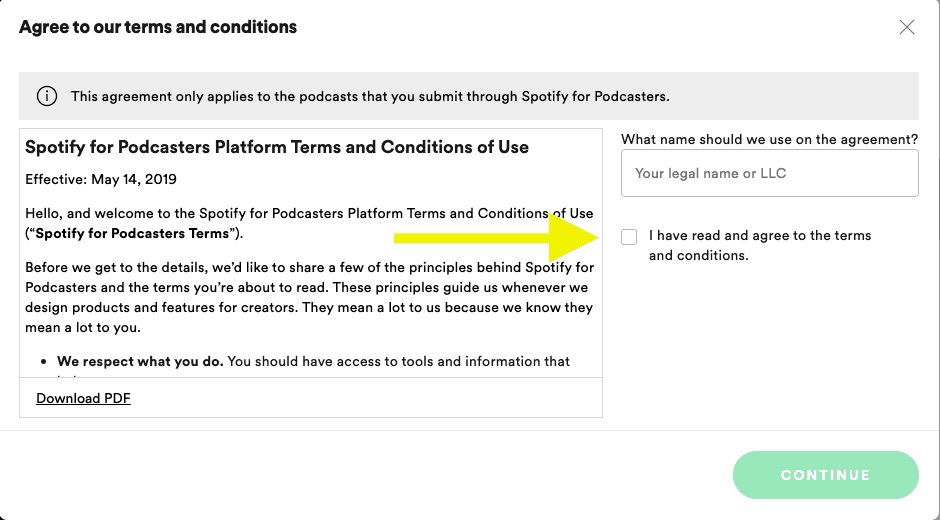This screenshot captures an agreement page on a website featuring the "Spotify for Podcasters" terms and conditions. The page includes a white header with prominent, bold black text at the top left that states: "Agree to our Terms and Conditions." On the top right, a medium gray "X" symbol is clearly visible as a close button.

Below this header, the page features a light gray rectangle with a black "eye" icon encircled in black on the left side. Adjacent to this icon, black text reads: "This agreement only applies to the podcast that you submit through Spotify for Podcasters."

The main content area is divided and enclosed by a thin light gray outline. In the top-left section, bold black text announces: "Spotify for Podcasters Platform Terms and Conditions of Use." Subtext in smaller gray font indicates: "Effective May 14, 2019." The introduction welcomes visitors and introduces the terms: "Hello and welcome to the Spotify for Podcasters Platform Terms and Conditions of Use."

Beneath a left-justified line of bolded black text within parentheses—"(Spotify for Podcasters Terms)"—a paragraph in gray font outlines the guiding principles of the terms, emphasizing their importance: "Before we get to the details, we'd like to share a few of the principles behind Spotify for Podcasters and the terms you're about to read. These principles guide us whenever we design products and features for creators. They mean a lot to us because we know they mean a lot to you."

Following this introduction, a bolded bullet point states, "We respect what you do." To the right, gray text begins a sentence: "You should have access to tools and information that," but the rest of the text is obscured.

The page is further divided by a thin light gray line. Beneath it, another white rectangle contains underlined black text on the left side that reads: "Download PDF."